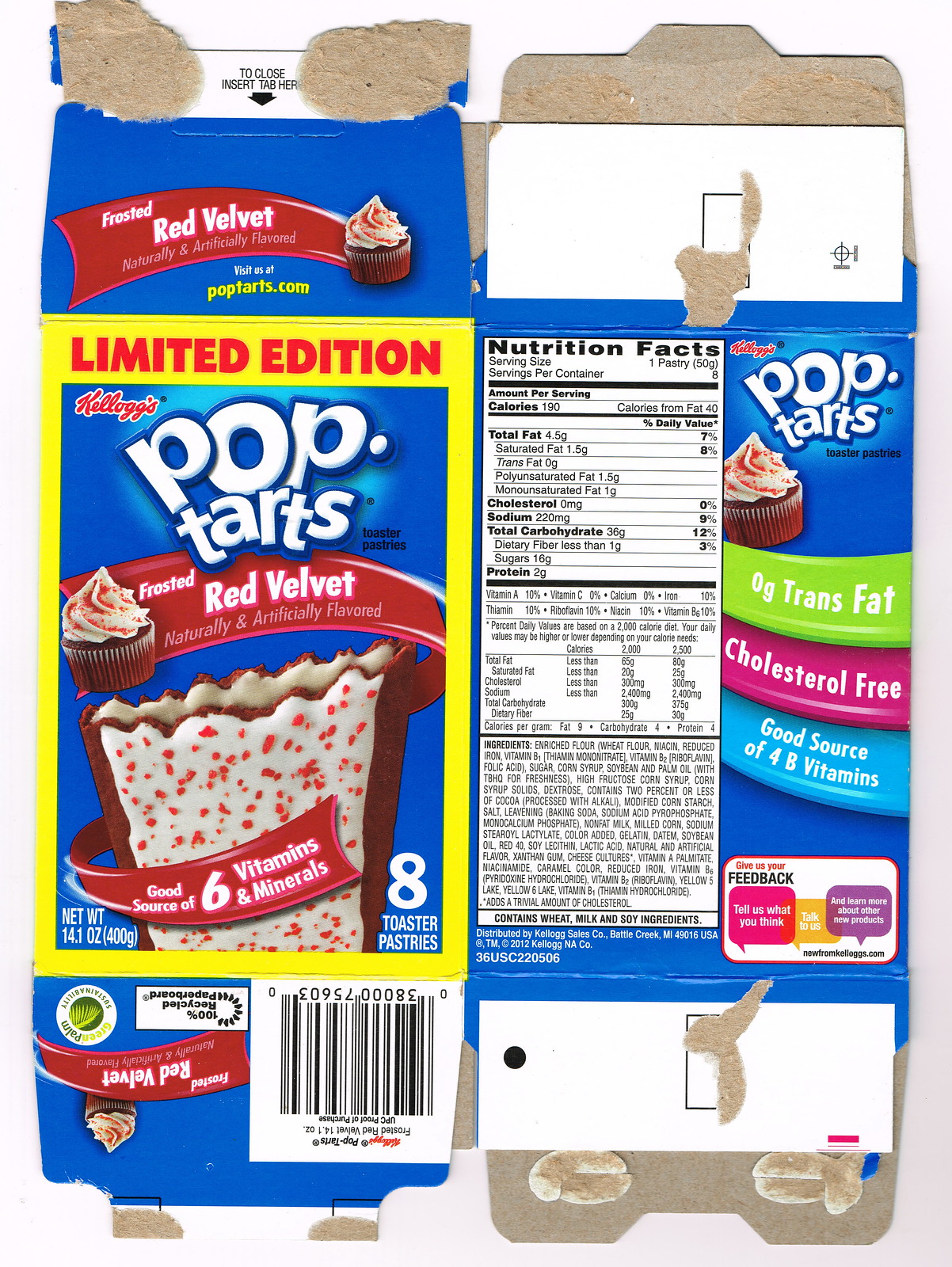This photograph showcases a flattened and empty Pop-Tarts box, revealing both the front and back panels of the packaging. The box, primarily blue, is torn at the top and bottom flaps, exposing remnants of glue on the right side and ripped cardboard on the left. The front side, outlined in bright yellow, features "Limited Edition" in red text, along with the iconic Kellogg's Pop-Tarts logo in white. Below this, a red ribbon wider on the left displays "Frosted Red Velvet, Naturally & Artificially Flavored." The central image is a digital rendering of the Red Velvet Pop-Tart, characterized by its dark red exterior, white frosting with red speckles, and a cream-filled interior. 

A small red velvet cupcake with white frosting and red sprinkles accompanies the product image. Both "Good Source of Six Vitamins and Minerals" and "Eight Toaster Pastries" are declared, with the latter located in the bottom right corner. The leftmost part of the back panel features a detailed nutritional fact panel against a white background, stating information such as 190 calories per serving, 4.5 grams of fat, and 16 grams of sugar, among other specifics. Adjacent to this are various digital banners: a green one announcing "Zero Trans Fat," a pink one stating "Cholesterol Free," and a blue one emphasizing "Good Source of Four B Vitamins." This side also reiterates details about the product flavor and nutritional benefits, accompanied by a smaller image of a red velvet cupcake akin to the Pop-Tart flavor. The overall presentation balances detailed visual and textual content, making the packaging information accessible and visually engaging even in its flattened state.